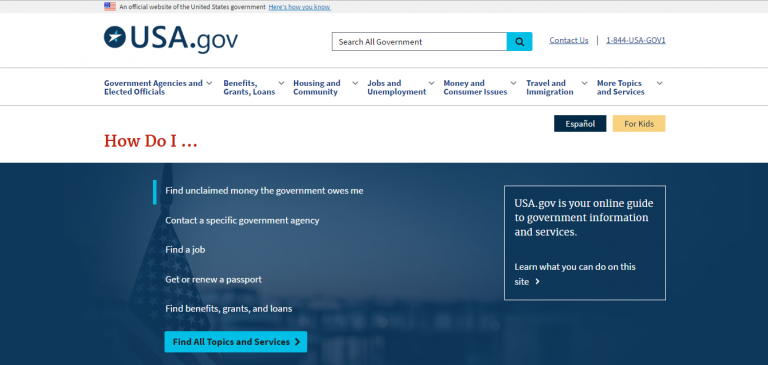The homepage of USA.gov features a clean and informative layout designed to provide users with easy access to a variety of government resources. At the top center, a prominently placed search bar invites users to quickly find the information they need. The header includes a contact number, 1-844-USA-GOV1, for direct assistance.

The main navigation menu is organized into comprehensive categories: Government Agencies and Elected Officials, Benefits, Grants, Loans, Housing and Community, Jobs and Unemployment, Money and Consumer Issues, Travel and Immigration, and More Topics and Services. Each category includes dropdowns offering further sub-sections.

The primary banner reads "How do I," followed by a quick access menu to facilitate tasks such as finding unclaimed money, contacting specific agencies, locating job opportunities, obtaining or renewing passports, and understanding available benefits. Users can also opt to explore all topics via a dedicated link.

Below the banner, text highlights the purpose of the site: "USA.gov is your online guide to delivering information and services. Learn what you can do on this site." This message is enclosed in a small informational box.

The design features a blueish background with an upright American flag that adds a touch of national identity. At the very top of the site, a disclaimer states, "The unofficial website of the US government. Here's how you know," accompanied by a link explaining its authenticity.

Overall, USA.gov serves as a centralized online resource hub for a wide range of federal government services and information.